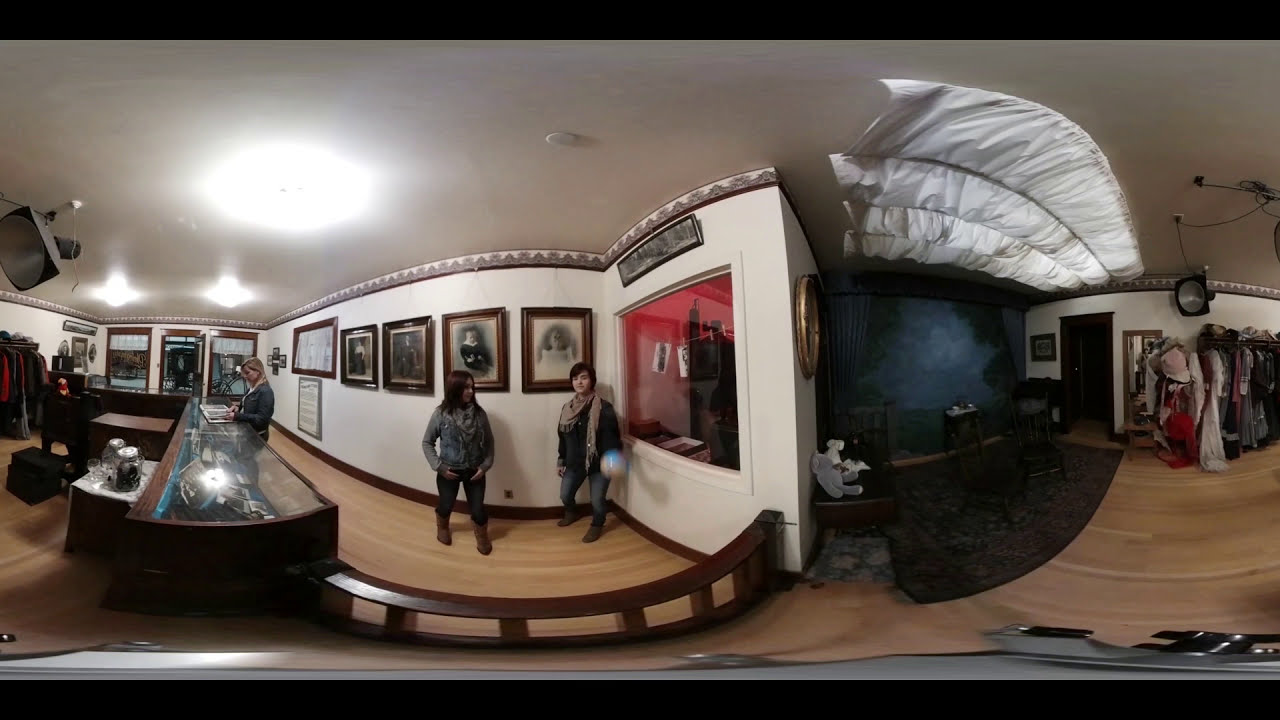The image depicts an intricately detailed room with a blend of gallery and business elements, possibly a photography studio or an art showroom. On the left side, the focus is drawn to two people standing near a series of framed portraits and artwork adorning the walls, all illuminated by an overhead light. A woman is seen either working or browsing through a book at a glass table, adding depth to the scene.

The floor is a light tan slatted wood, complemented by a Persian rug with chairs placed upon it. In the center bottom of the frame, a kneeling or sitting bench provides a break in the spatial layout. The right side of the room features a dark blue wall serving as a backdrop scattered with green plants, enhancing the aesthetic appeal. This area also includes a photo booth setup and a collection of clothing on racks, possibly costumes from different historical eras.

A white drape on the ceiling suggests a light diffuser, consistent with the setup of a portrait photography studio. A display case with brown wood trim and glass sides can be seen, adding to the business-like ambiance with its curated display. The main colors in the room are varied yet harmonious, featuring shades of brown, white, and red. Additional details include a smoke detector on the ceiling, reinforcing the meticulous attention given to the setting. This eclectic mix creates a visually engaging space where visitors can appreciate both the artistic and functional elements of the environment.